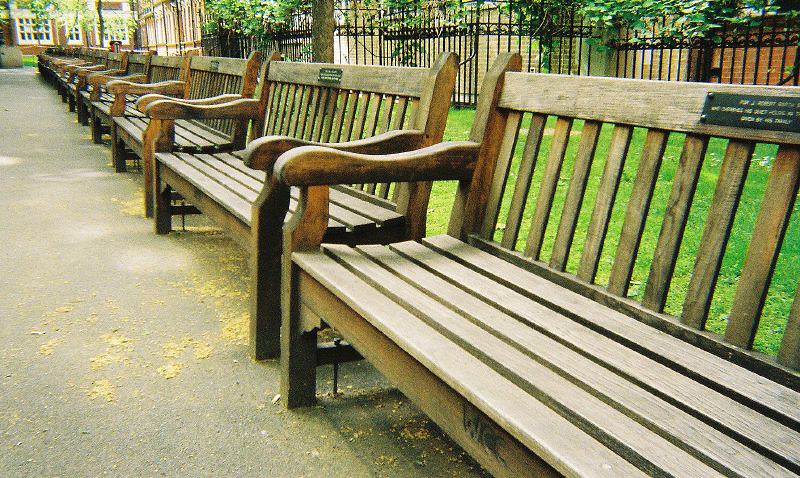The photograph captures a long row of weather-worn wooden park benches, extending diagonally from the lower right corner to the back left, creating a sense of depth as they fade into the distance. Each bench, composed of light brown wood with five horizontal slats for seating and vertical slats for the back, features slightly curved armrests and straight legs. A black plaque, possibly a dedication or memorial, is mounted at the center top of each bench, though the inscriptions are not legible. The benches rest on an asphalt walkway, which is sparsely scattered with fallen yellow and green leaves, suggesting a springtime setting. Beneath some benches, there are signs of moss and possibly bird food. Behind the benches, a narrow strip of well-maintained grass leads to a wrought iron fence adorned with lush green vines. Beyond the fence, several brick buildings in varying shades—from deep red with white-trimmed windows to lighter tan bricks—punctuate the background. The scene, illuminated by daylight, offers a tranquil snapshot of a park or possibly a college campus quad.